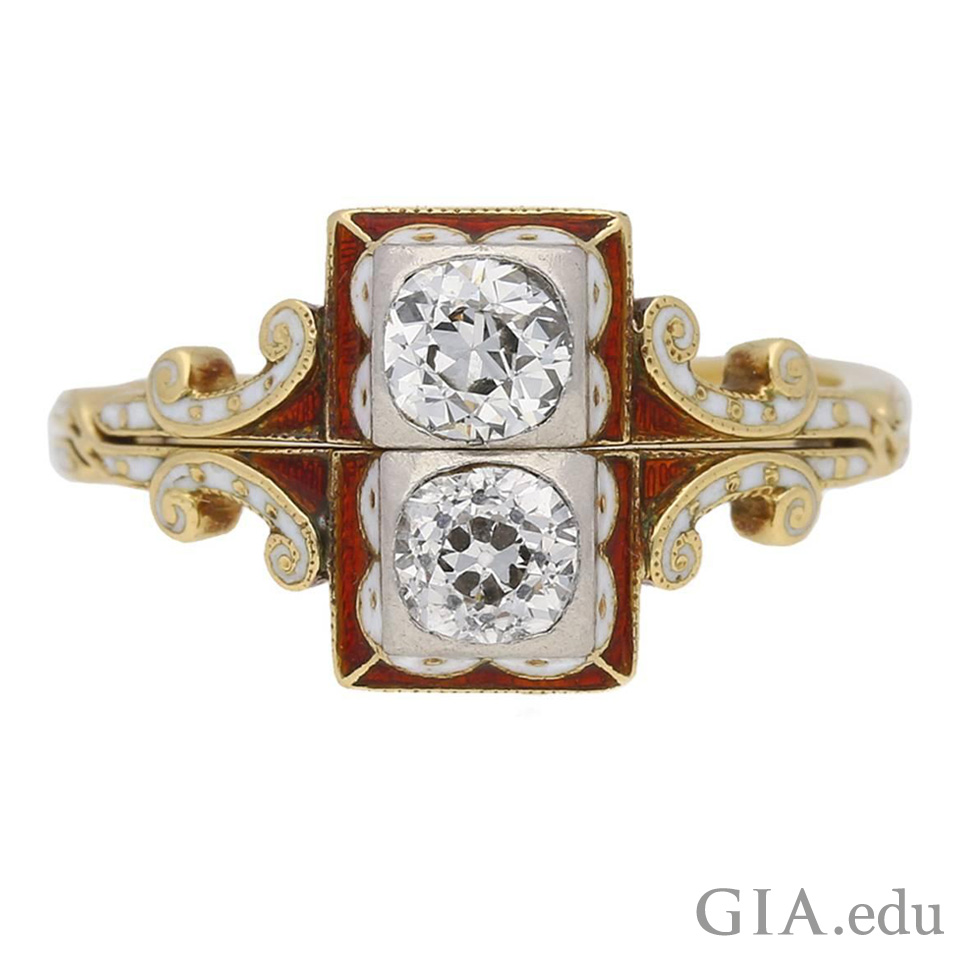This is a detailed and color photograph of an antique, custom ring, likely used for advertisement purposes, set against an all-white background. The ring boasts a captivating design featuring a central element composed of two stacked squares. Each square has an intricate layout: a red enamel border with gold elements, a silver interior, and a centrally embedded brilliant round diamond. There are notable differences in the diamond cuts, emphasizing the unique nature of each stone. Along the band, the ring displays intricate swirling motifs in gold that resemble the letter "C," interspersed with white enamel dots running through the center. This detailed craftsmanship extends around the entire ring. The photograph also includes the text "GIA.edu" at the bottom right corner, suggesting an association with the Gemological Institute of America. The staging of the image leaves some ambiguity about whether the ring is reflected on a shiny surface or if it consists of multiple parts. There are no people visible in this meticulously composed advertisement-like photograph.